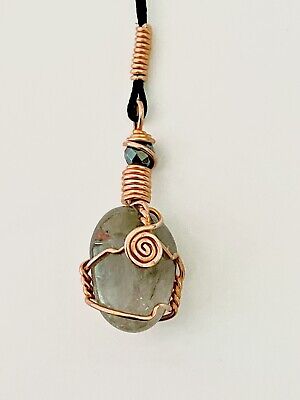This image showcases a detailed close-up view of a jewelry pendant. The pendant features an oval-shaped stone with a grayish-beige hue, resembling a dusty or dirty white color. The stone is elegantly encircled by shiny copper wire, which wraps around it multiple times. At the center of the stone, there is a decorative spiral of copper wire. This wire continues upwards, twisting into an intricate design at the top, creating a loop through which a black string is threaded. The black string is attached to a copper hook at the top. The background appears to be an oxide or cream-colored surface, adding contrast to the pendant’s design. Additionally, golden rings and green gemstones can be seen as part of the pendant or its surrounding decor. The overall appearance suggests that the pendant is an artifact or locket, meticulously crafted with intricate copper wire detailing and adorned with green gemstones.